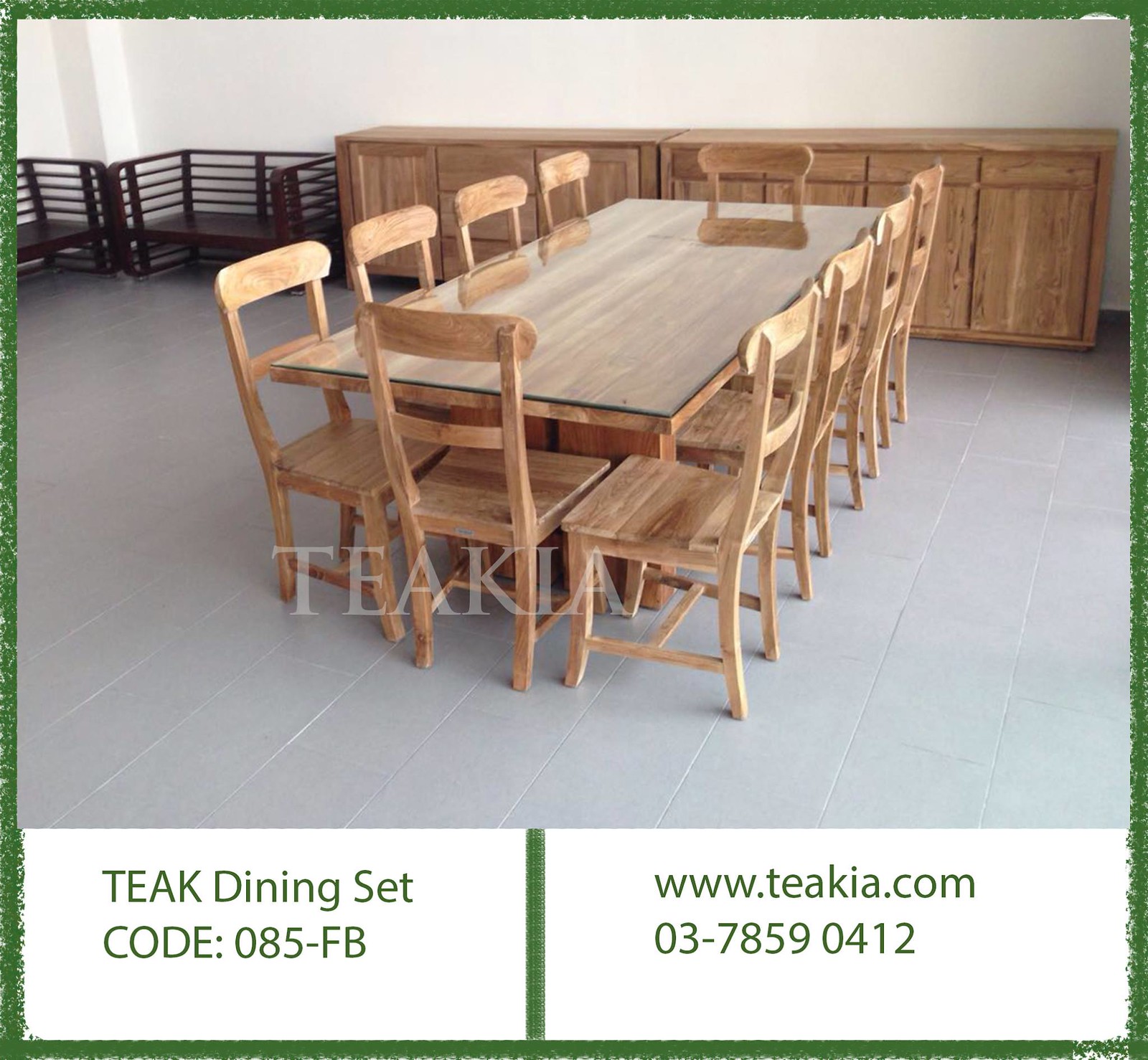This is an advertisement for a teak dining set with the code 085-FB. The central image showcases a large, tannish-brown teak dining table topped with glass, surrounded by ten matching wooden chairs—four on each side and one at each end. The set is placed on gray flooring, exuding a refined, cohesive look. In the background, there is a teak cabinet with four doors and small drawers above them, alongside a second cabinet featuring two doors and three middle drawers, both accentuating the dining set. Additionally, there are black stand-like structures on the left that are empty. The image features the text "T-E-A-K-I-A" in white, centrally placed over the furniture. Below, a green-bordered section reads "Teak Dining Set, code: 085-FB" on one side and "www.teakia.com, 03-7859-0412" on the other.